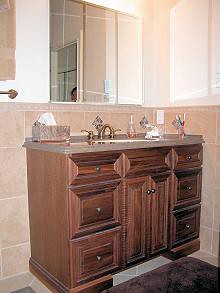The photograph captures the interior of an elegantly designed bathroom. At the center of attention is a single sophisticated sink with an ornate marble countertop. The sink is adorned with gold spigots and dual side handles for hot and cold water. The backdrop features beautifully tiled walls in a delicate peachish rose color. Mounted above the sink is a mirror which reflects parts of the room, revealing a standing shower and a window.

Adjacent to the sink, a neatly hung hand towel adds a touch of convenience. A Kleenex box is situated on the left side of the sink. The bathroom floor is graced with a new-looking brown rug, enhancing the room's inviting ambiance.

The wooden cabinetry beneath the sink boasts an intricate design, comprising six drawers—three on each side—and a faux drawer at the top center, accommodating the sink's plumbing. Additionally, there are two cupboards with brass handles that open outwards, completing this luxurious and thoughtfully arranged bathroom space.